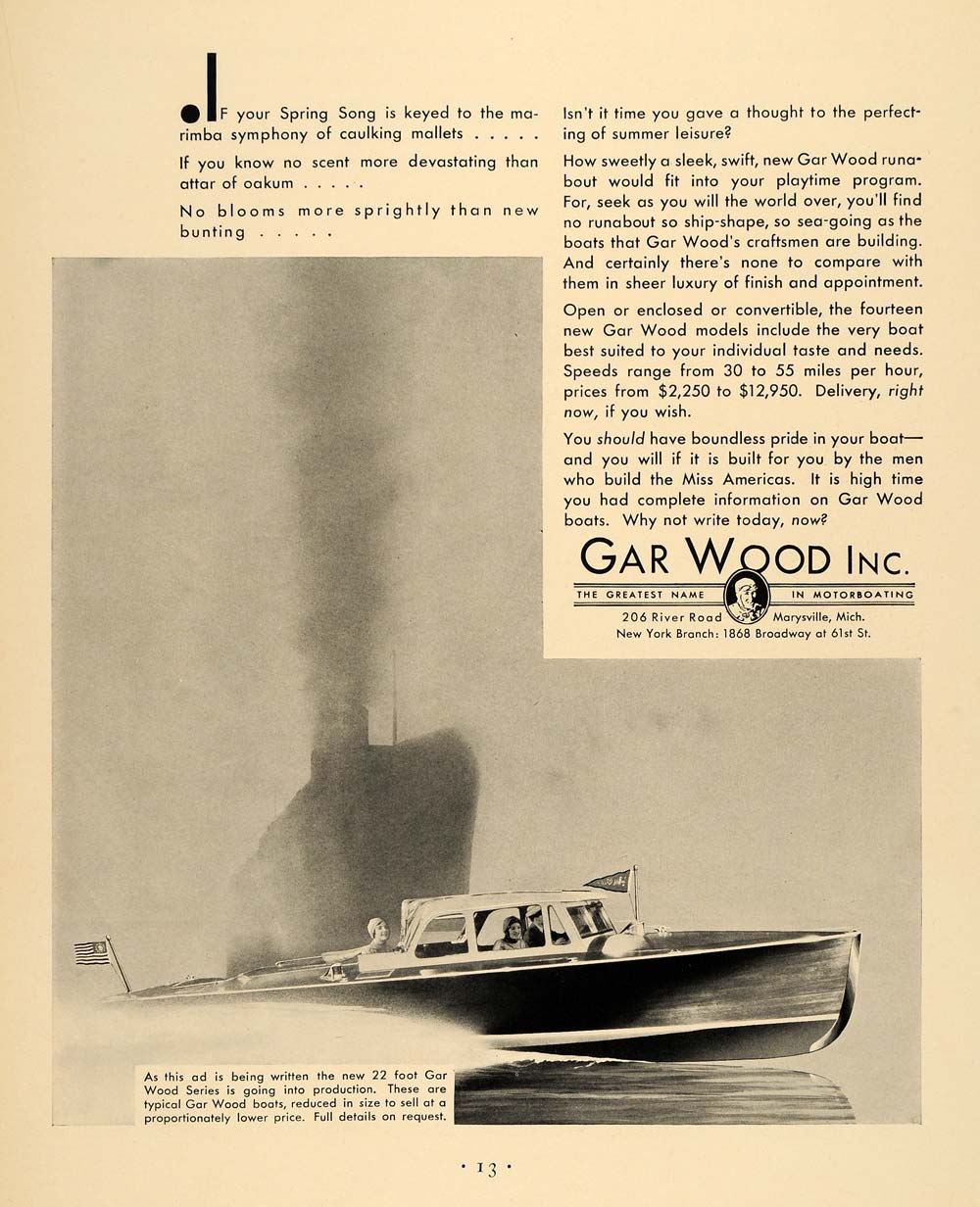This sepia-toned page, likely from an early 20th-century magazine or newspaper, features an advertisement for Gar Wood Inc., touted as the greatest name in motor boating. The image is a detailed hand-drawn illustration of a 15 to 22-foot speedboat with a covered cabin and an open back, proudly displaying a stylized United States flag. This boat speeds through the water in front of a large, silhouetted steamship in the background. The advertisement text, occupying the top half of the page in two columns, poetically invites readers to consider the Gar Wood runabout for enhancing their summer leisure time. It highlights the craftsmanship, sea-worthiness, and luxury of the 14 new models, which cater to individual preferences and range in speed from 30 to 55 miles per hour, priced between $2,250 and $12,950. Delivery is available immediately. The ad, set against the backdrop of an intersection between playful and elegant imagery, underscores the renowned quality and sophistication of Gar Wood boats, with contact details provided for further inquiries at the 206 River Road headquarters in Maryville, Michigan, and a New York branch office.